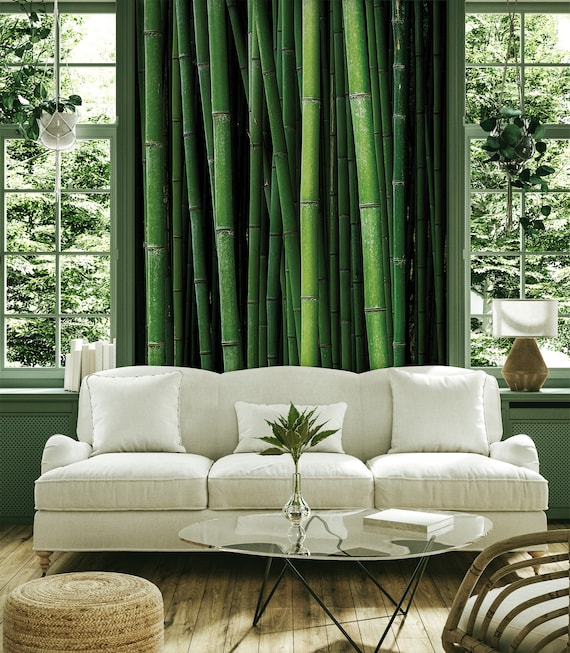The image depicts a meticulously designed living room characterized by a nature-inspired theme. The focal point is the back wall, adorned with large, green bamboo stalks stretching from the floor to the ceiling, likely a detailed wallpaper or a wall decal, anchoring the room's natural aesthetic. Flanking this bamboo feature are two tall, identical windows allowing views of lush green trees outside. Each window has a hanging white pot with verdant, leafy vines cascading down, adding to the indoor greenery.

Centered against the bamboo-decorated wall is a light-colored, almost white couch, adorned with three white throw pillows and flanked by additional larger white cushions on both ends. Below the windows, the wall is painted a dark green, blending seamlessly with the forest theme.

In front of the couch rests a glass coffee table with sleek black metal legs. This table holds a clear vase with a single green plant stalk and a white book, continuing the room's clean and organic motif. The floors are natural wood, complementing the earthy decor.

To the left of the couch, a tan woven ottoman provides additional seating. On the front right, there is the corner of a chair characterized by its brown wicker-like frame and a white cushion. This serene yet elegant living space blends clean lines and comfortable furnishings with lush, nature-heavy elements, creating a modern, tranquil oasis.